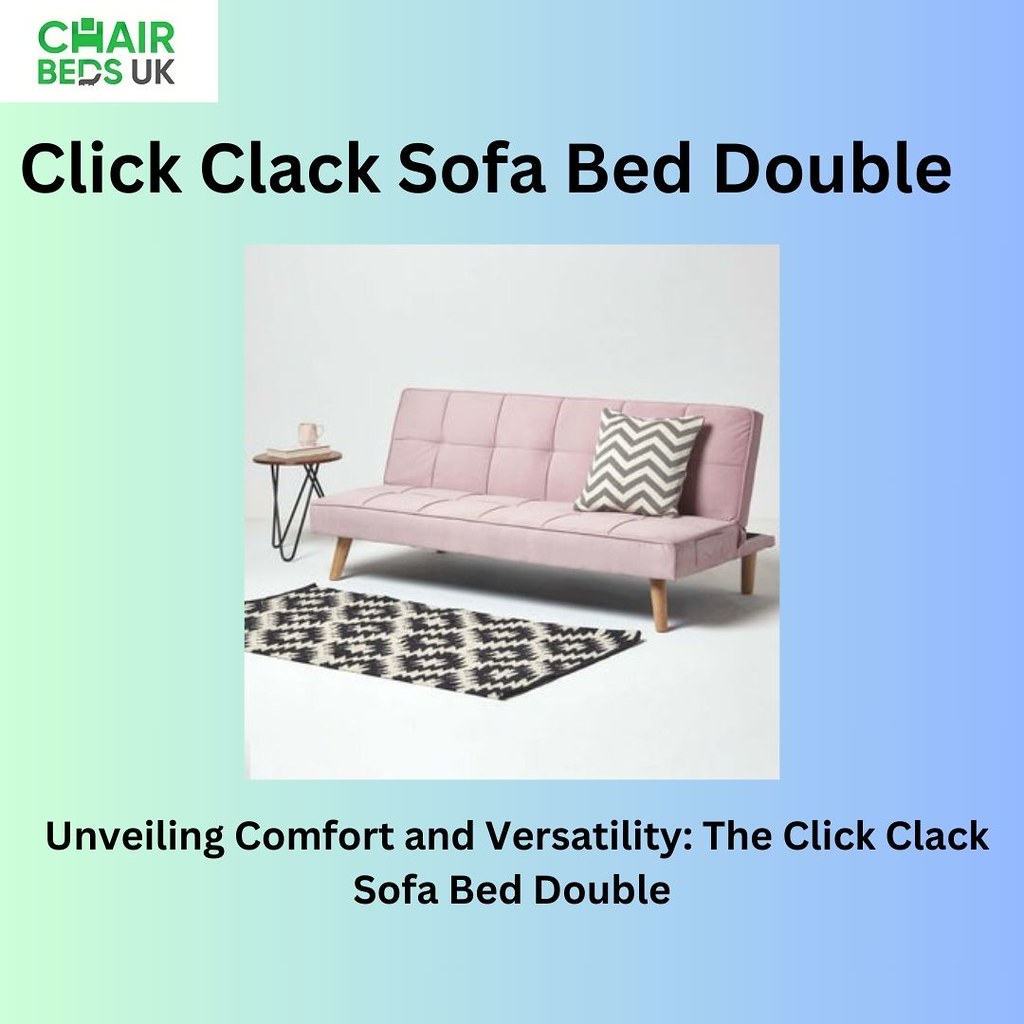The image features a light pink futon with wooden legs against a white background. The futon has a white pillow adorned with green chevron zigzag lines on the right side. It sits atop a white throw rug with a diamond pattern. In the foreground, there is a brown side table with a book and a white mug, supported by black and white legs. The entire background transitions from a light pastel green on the left to a light pastel blue on the right, providing a subtle gradient effect. Text on the upper left corner reads "Chair Beds UK," with the H stylized as a chair and the D as a lounge chair. Bold black text across the top declares "Click Clack Sofa Bed Double." Below the futon image, additional black text reads "Unveiling Comfort and Versatility" followed by "The Click Clack Sofa Bed Double." This composition appears to be an advertisement for a versatile and comfortable sofa bed.